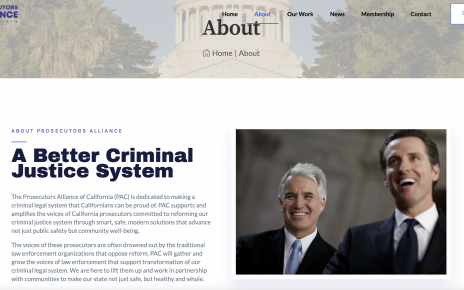The webpage features a predominantly white background. At the top of the image, there is a rectangular section that appears partially cut off. In the top left corner, there is a glimpse of purple text, with only the letters "NCE" visible, suggesting the rest is cut off. This top section also includes a background image showing a few trees and what appears to be the dome of a capitol building.

Below this, a navigation menu includes the following options in black text: "Home," "About," "Our Work," "News," "Membership," and "Contact." The "About" option is highlighted in blue to indicate it is currently selected. Underneath this menu, in larger black text, is the heading "About."

Further down is a breadcrumb trail with a Home icon, followed by the text "Home / About." Directly beneath this, set against a white background, there is an image towards the bottom featuring two smiling white men. Both are dressed in black suits; the man on the left has dark hair and is wearing a blue tie, while the man on the right has gray hair and a black tie.

To the left of this image, purple text reads "About Prosecutors Alliance." Below that, in large black text, is the phrase "A Better Criminal Justice System." Below this heading are several lines of smaller black text that are difficult to read and make out clearly.